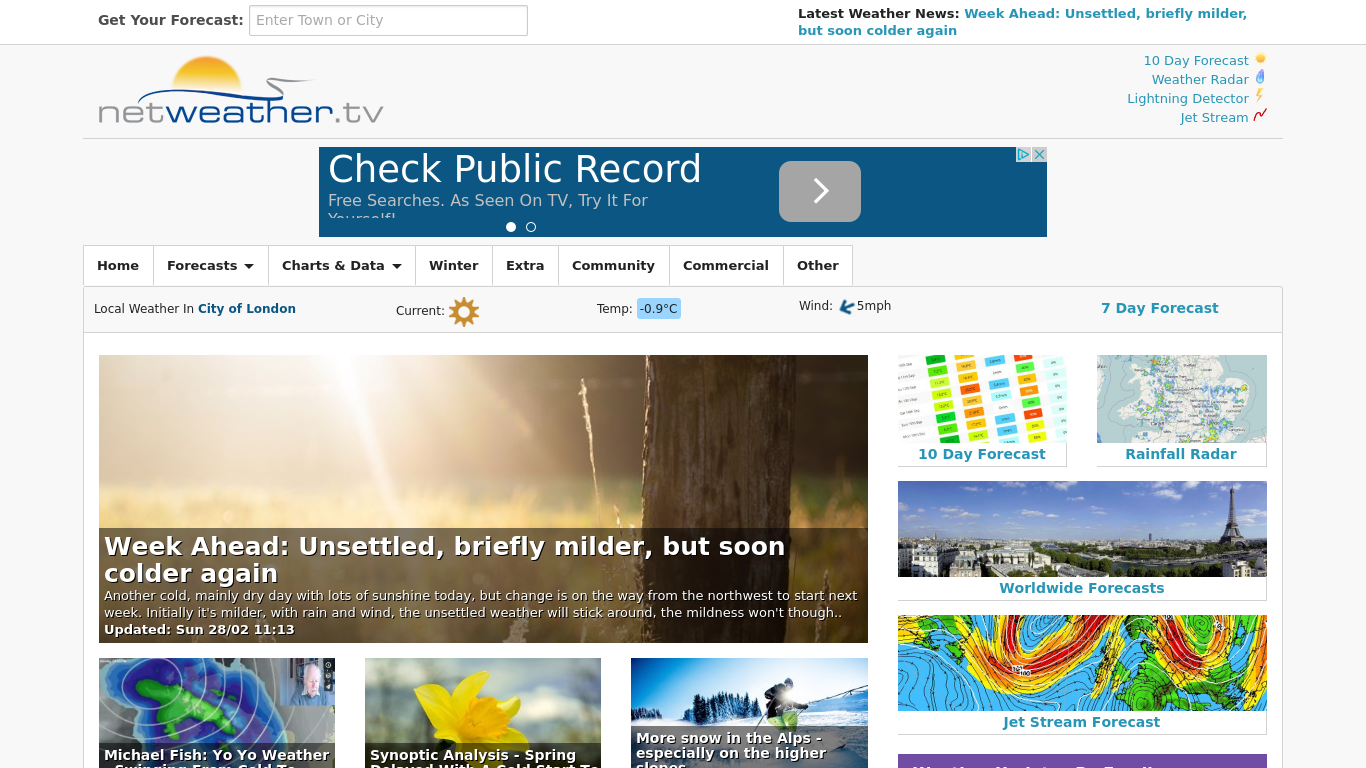The screenshot captures a webpage from a weather forecasting website. At the top, there's a white bar featuring "Get your forecast" in black font on the upper left. Adjacent to that is a search rectangle where users can type in their town or city. On the upper right, it reads "The latest weather news:" in black font, followed by a weather update in light blue font: "Week ahead; unsettled, briefly milder, but soon colder again."

Beneath the top bar, the page content begins. On the upper left, the site branding shows "netweather.tv" accompanied by an icon of a setting sun above the text. On the upper right, there are navigation links: "10-day forecast, weather radar, lightning detector, jet stream."

Directly below, a banner ad says, "Check public record, free searches as seen on TV, try for yourself" within a purple backdrop. The main navigation follows, offering links to "Home, Forecast, Charts and Data, Winter, Extra, Community, Commercial, and Other."

The central section of the page highlights the local weather in the City of London. It shows the current weather condition as sunny, indicated by a sun icon, and lists the temperature as 0.9°C.